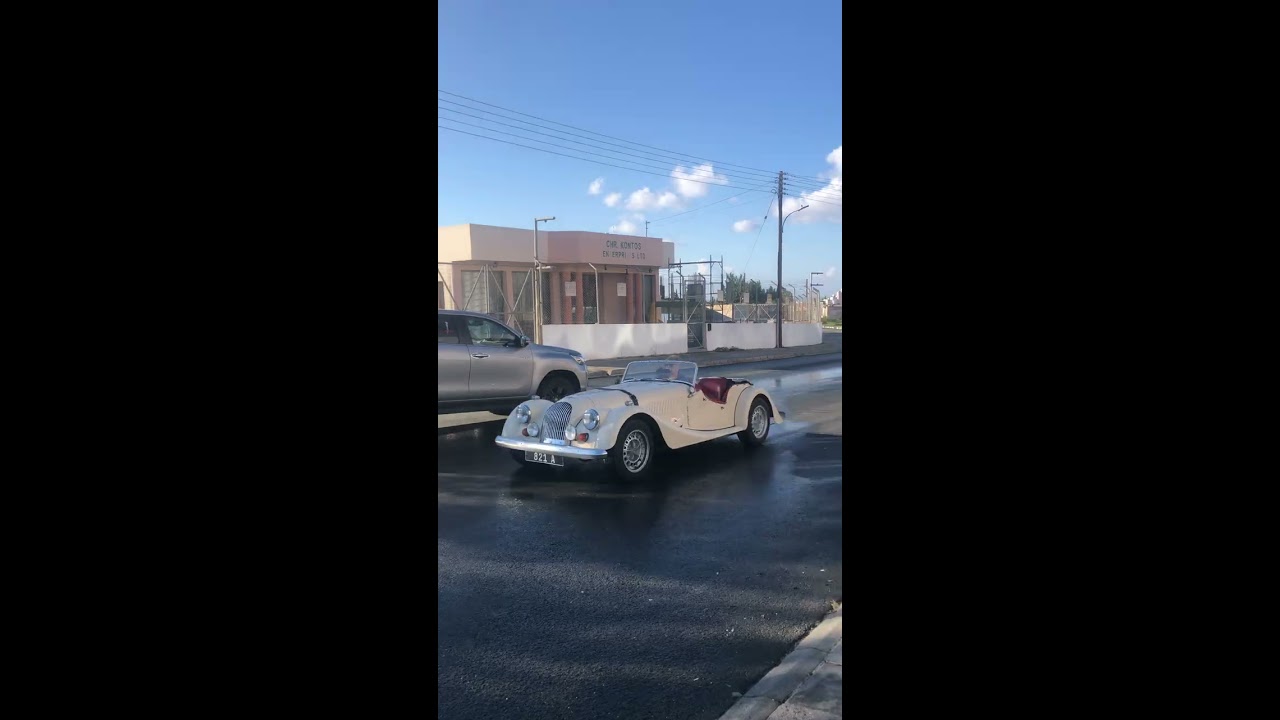The photo captures a charming scene outside on a sunny day, with a clear blue sky accented by a few white clouds. Centered in the image is a beautifully maintained vintage white convertible, likely from the 1940s or 1950s, showcasing its timeless design and elegance. The car's dark red leather seats gleam in the sunlight, and its roof is down, exposing the detailed interior. The sleek, elongated front is adorned with a large rectangular grille, round silver lights, and a chrome bumper. Its curvy wheel arches add to the car's classic allure. A single individual is driving the car, which is positioned on a smooth blacktop, possibly a city street. On the right side of the image, a modern silver pickup truck contrasts with the vintage car, and a pink building can be seen on the roadside, enhancing the nostalgic atmosphere. Power lines crisscross above, adding a touch of urban scenery. The driver is situated on the right side of the vehicle, indicating the location might be outside the US.